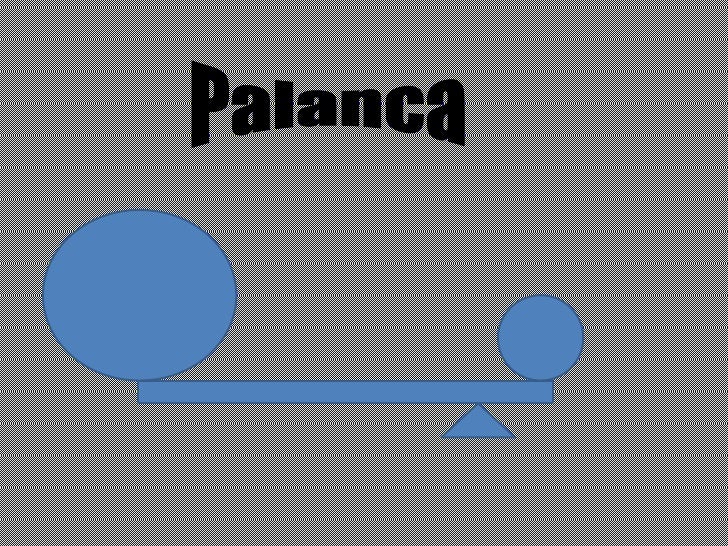This image appears to be a meticulously designed advertisement or poster, possibly generated by a computer, with a minimalist gray background subtly textured with fine black and white dots forming a slatted window-like pattern across the entire surface. Dominating the top of the image, the word “Palanca” is presented in an eye-catching black font that gives a cinemascope-like visual effect, with the first letter 'P' capitalized and the rest in lowercase, wrapping slightly around. Below the text, occupying the bottom half of the image, is a striking geometric diagram resembling a teeter-totter or lever mechanism. This design features a wide, thin blue rectangle representing the lever. On the left end of this lever is a large blue circle, while on the right end is a smaller blue circle. The lever is balanced on a blue triangle, the fulcrum, situated near the smaller circle on the right end, emphasizing the imbalance created by the differing sizes of the circles.